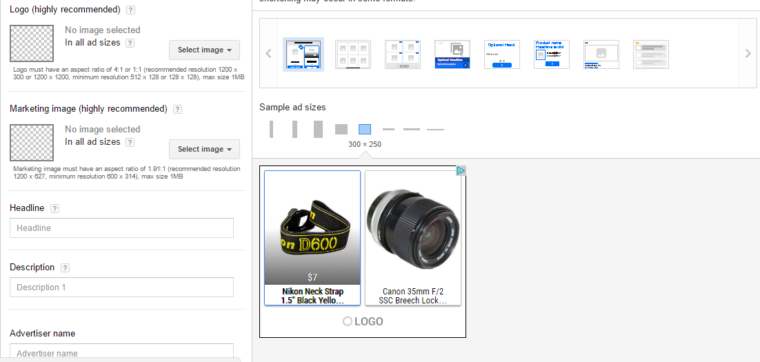This image is a screenshot of a photo editing program with a predominantly white background and black and gray text. The left side features a vertical menu with five distinct options, with the top two marked as "highly recommended." 

1. **Logo (Highly Recommended):** A checkerboard placeholder indicates no image has been selected for all ad sizes. A drop-down menu labeled "Select Image" is next to it.
2. **Marketing Image (Highly Recommended):** Similarly, this option also has a checkerboard placeholder and a "Select Image" drop-down menu.

Below these options, there are three text fields labeled:
- **Headline**
- **Description**
- **Advertiser Name**

The right side of the screenshot is partially cut off at the top, making some text unreadable. However, it displays a series of eight thumbnails, possibly screenshots of different web pages. This section is labeled "Sample ad sizes," with the currently selected size being 300 by 250 pixels.

Beneath these thumbnails, two side-by-side product images are shown:
- **Camera Strap:** Priced at $7, labeled "Nikon Nexstrap 1.5 inch black yellow."
- **Camera Lens:** Labeled "Canon 35mm f/2 SSC breach lock."

This detailed layout suggests the program is designed for creating advertisements, providing both image and text customization options.